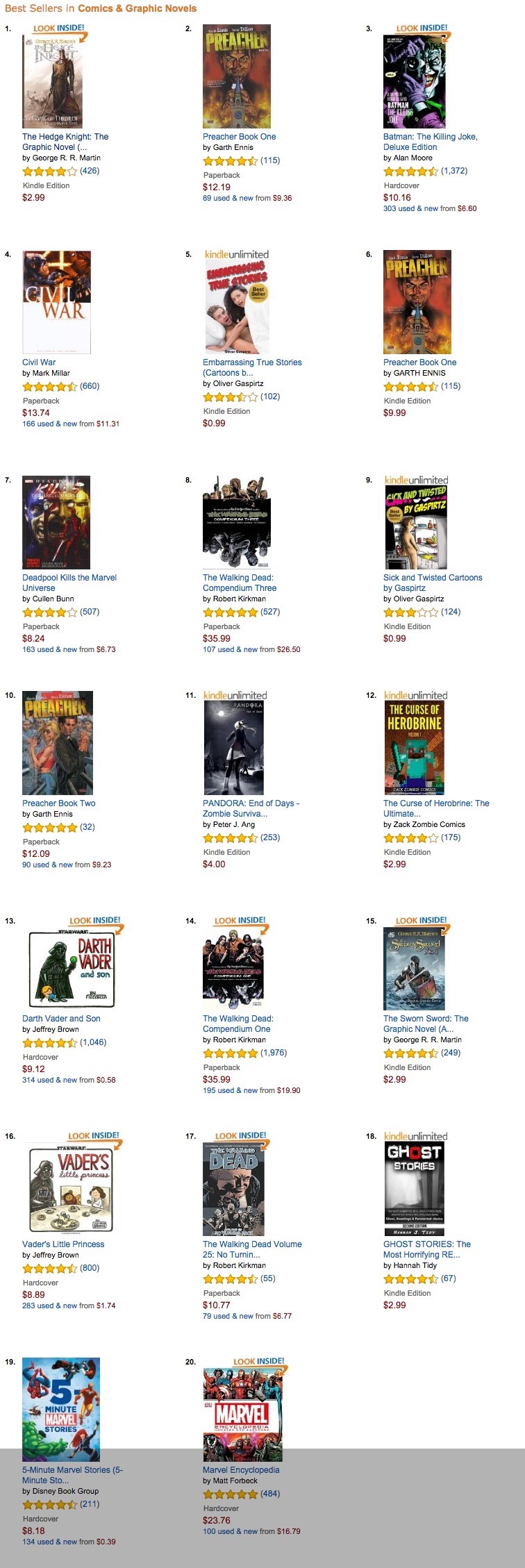This screenshot showcases a selection of 18 highly-rated video games and graphic novels, each boasting five-star reviews. Among these featured titles is the "Batman: The Killing Joke, Deluxe Edition," available for Kindle. The items are described with detailed reviews highlighting both their strengths and weaknesses. The graphic novels offer a "Look Inside" feature, allowing potential readers a glimpse into the content. The diverse mixture of video games and graphic literature presents a rich array of entertainment options for enthusiasts.